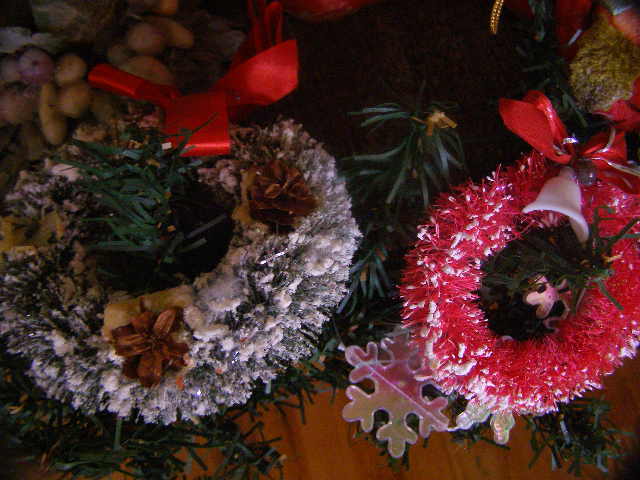This image features a close-up view of two Christmas tree ornaments set against a wooden floor scattered with pine needles. Both ornaments are wreaths. The one on the left is white with a snow-dusted texture, adorned with small pine cones and a red bow. Pine needles poke through its open center, adding to the festive feel. The wreath on the right is red, also snow-dusted, and it features a red bow at the top with a small white bell suspended below. Radiating around the red wreath, pine needles emerge through the open center. In the background, the wooden surface transitions to a darker, mostly black backdrop with a hint of other Christmas decorations, including a silvery snowflake-like object in the upper right corner and possibly some additional ornaments partially visible. This real-life photograph captures the detailed textures and colors of the holiday ornaments, creating a warm and festive scene.